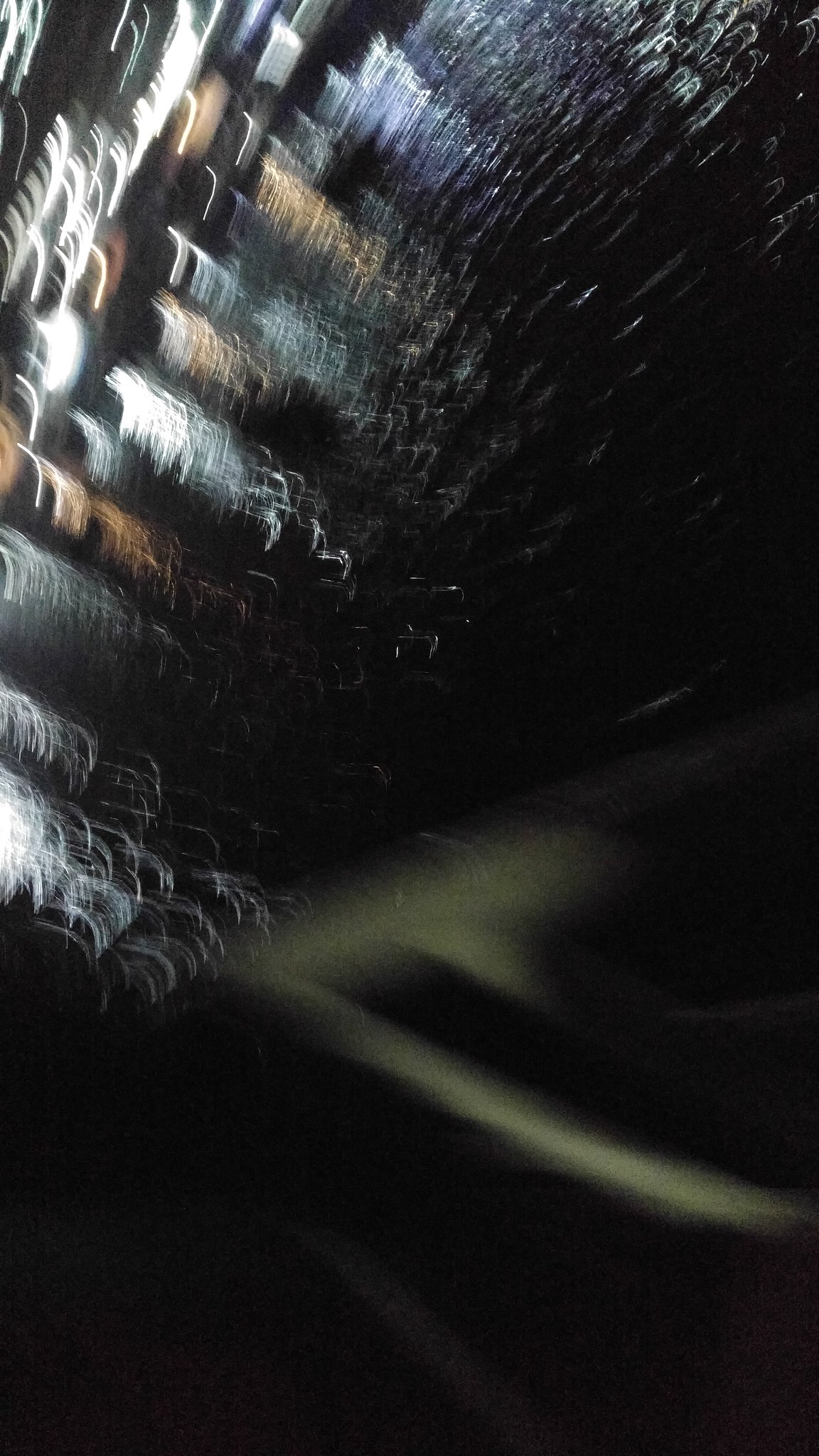This heavily blurred and abstract close-up photograph features a predominantly black rectangle with a bottom portion that is smoother and shows subtle wave-like textures. The image is likely a result of long exposure, capturing what seems to be feathers or hair in motion, leading to a confusing yet intriguing visual. The upper left portion is filled with tiny white separations—possibly feathers or strands of hair—that arc towards the upper right corner. These white elements, along with hues of burnt orange, cream, and a pale yellow, contribute to the chaotic yet captivating detail of the piece. The image has no text and gives a modern art impression, with some viewers interpreting it as moving lights captured against a dark backdrop, while others see natural elements like feathers or hair. The dominant colors are black, white, and a mix of yellow or copper tones, creating a curious and mystifying composition.